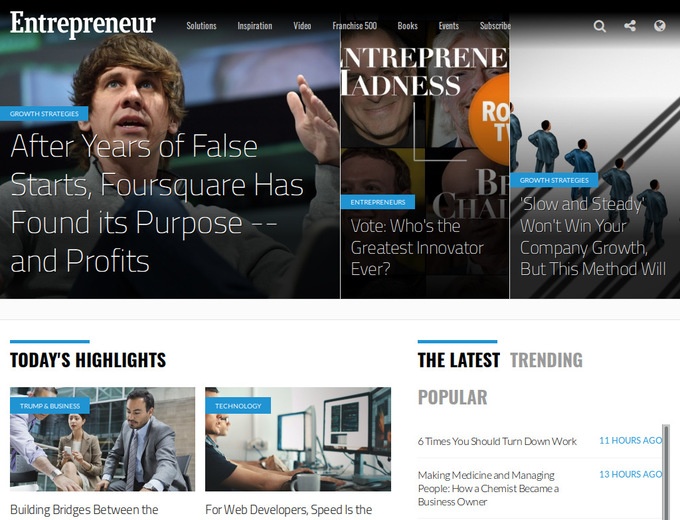Here's a detailed and cleaned-up version of the caption:

"This image captures several articles featured on a digital platform for Entrepreneur magazine. In the upper left corner, a prominently displayed article shows a white man wearing a long-sleeved shirt, with his mouth slightly open, looking upwards. The title 'After Years of False Starts, Foursquare Has Found Its Purpose—and Profits' is presented under a blue banner labeled 'Growth Strategies,' while 'Entrepreneur' is inscribed in white.

To the right, a partially visible second article reveals fragments of the words 'entrepreneur' and 'madness,' along with half of an orange circle containing the letters 'R, O, T'. It is topped with a blue banner that reads 'Entrepreneurs,' followed by the headline 'Vote: Who's the Greatest Governor Ever?' In the backdrop, there are indistinct images of men.

Further to the right, another article title is displayed under a blue banner that says 'Growth Strategies.' It features animated illustrations of men in blue suits gazing to the right, set against a background that fades from gray behind them to white in front of them. The headline 'Slow and Steady Won't Win Your Company Growth, But This Method Will' accompanies the visuals.

Below these articles, the section titled 'Today's Highlights' is marked in black text. One featured article bears a banner that says 'Trump and Business,' showcasing a man in a gray suit, a slightly Asian-looking woman in a tan suit, and another man whose face is partly obscured by the banner, all situated in an office environment. The text beneath reads 'Building Bridges Between the,' but it is cut off.

Additionally, there's an image of individuals at computers, labeled 'Technology' with the headline 'For Developers, Speed is the ...' visible on a blue banner. 

Lastly, on the right side, there's a list of the latest trending articles, including 'Six Times You Should Turn Down Work' posted 11 hours ago, and 'Making Medicine and Managing People: How a Chemist Became a Business Owner' posted 13 hours ago."